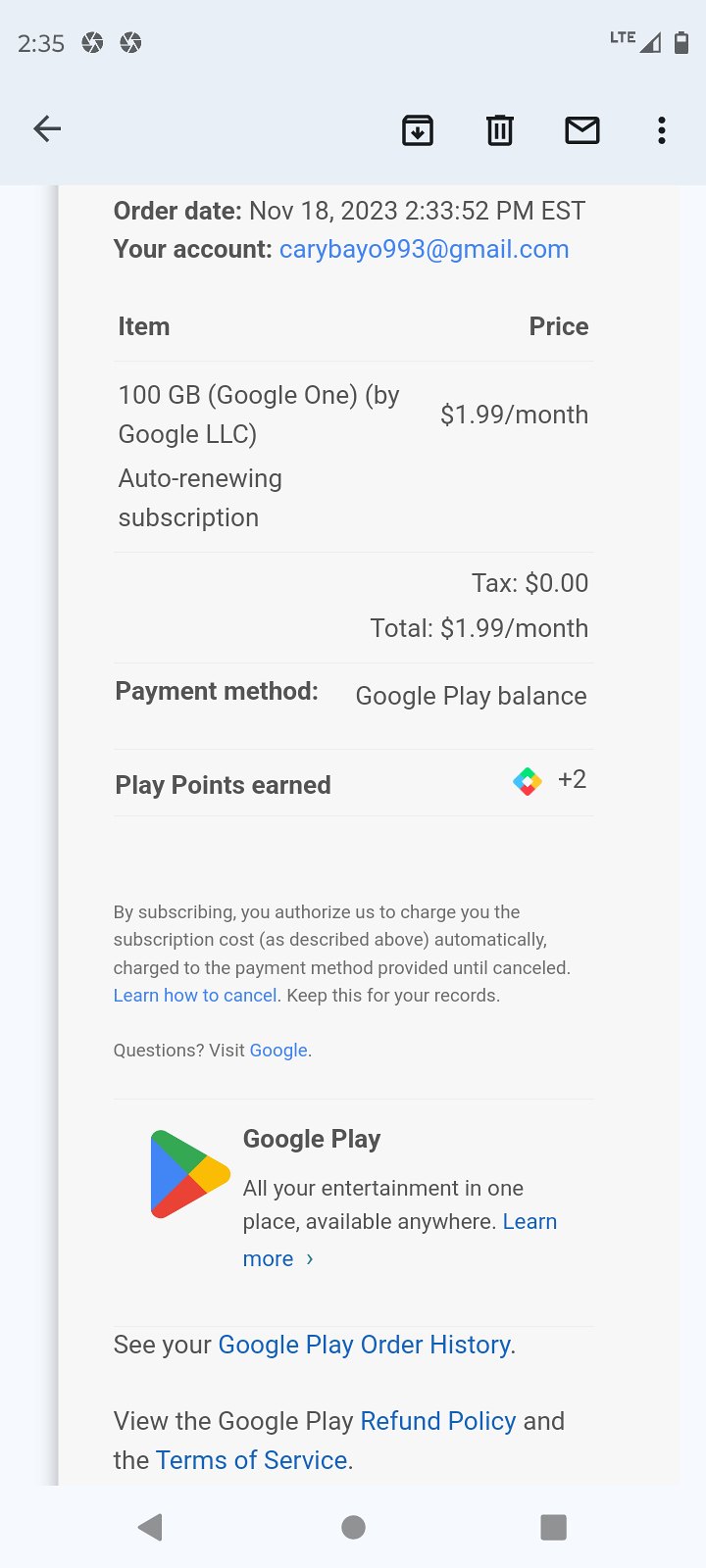**Caption:**

A digital receipt captured as a screenshot on a smartphone, displaying details of a purchase made using Google. The overall shape of the image is rectangular, with elongated left and right sides compared to the top and bottom. The background, header, and footer are gray, typical for a smartphone UI.

At the very top of the image, the status bar shows the current time as 2:35 PM. In the top right corner, "LTE," a half-filled triangle icon, and a battery icon indicate the phone's connectivity and battery status. 

Below the status bar, a gray arrow pointing left is visible on the left side of the screen, while the right side features a downward-pointing arrow inside a square, an outline of a gray trash can, and an envelope icon.

The main portion of the receipt is filled with black text detailing the purchase. It states:
- **Order Date:** NOV 18, 2023, 2:33:52 PM EST
- **Your Account:** karybayo993@gmail.com
- **Item:** 100GB Google One by Google LLC
- **Price:** [Not specified in the provided text]

The screenshot effectively captures the essential information of the transaction with the persistent elements of the smartphone interface.